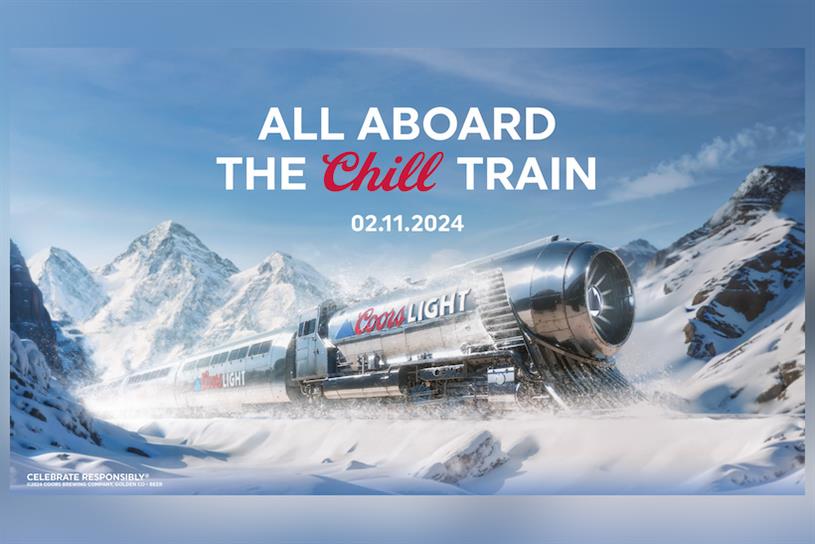This vibrant color illustration, in a landscape orientation, showcases a sleek silver train traveling from the left to the right side of the image. The front of the train highlights a circular opening housing a large vent fan, and beneath it, a curved tractor-like structure kicks up snow along the tracks. Emblazoned on the side of this leading car is the iconic red and white Coors Light logo, with "Coors" in elegant red script and "Light" in bold, all-capital letters. The adjacent car in the train also displays the Coors Light logo, while subsequent cars fade into the snowy backdrop. Above the train, the blue sky frames the bold white text, "All Aboard the Chill Train," followed by the date, "02.11.2024."

In the background, a majestic mountain range dotted with snow rises behind the train, complementing the snowy foreground bank. On the bottom left corner, white text urges viewers to "Celebrate Responsibly!" with an additional, yet unclear, line underneath. The overall scene, brimming with dynamic motion and vivid detail, effectively encapsulates the spirit of a chilly train journey through a wintry wonderland.